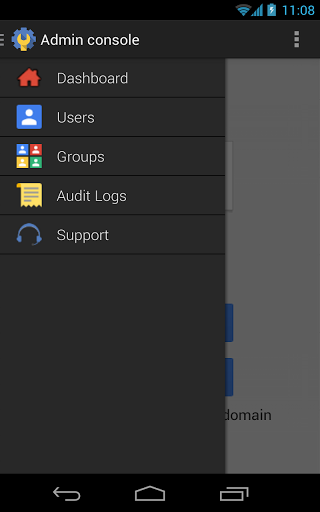The screenshot captures a vertical view of a phone's screen, showcasing several key features. At the top-right corner against a black banner, a row of blue icons represents various statuses. The Wi-Fi signal icon displays three out of four bars. Adjacent to it is the cellular service signal, showing full strength with four bars. The battery symbol follows, featuring a white lightning bolt indicating that the phone is charging. Next to these symbols is the time display, showing 11:08.

Centered under this banner is the "Admin Console" interface title in white letters. To its left is an icon of a cogwheel with a wrench superimposed, symbolizing settings. On the right side of the title, three small vertical squares act as a menu option.

Beneath the "Admin Console" title, a black rectangle signifies a clickable area. When accessed, it reveals an option screen with a dark background and white text. The topmost option is labeled "Dashboard," accompanied by a house icon on the left. Below it is "Users," indicated by a blue square with a person icon. The next option, "Groups," is identified by four small icons in blue, red, yellow, and green, each containing a person icon. "Audit Logs" comes next, marked with a yellow piece of paper with gray lines and jagged edges. The final option is "Support," represented by a headset icon.

At the bottom of the screenshot, three navigation icons are visible: an arrow pointing left, a house icon in the center, and two overlapping rectangles on the right.